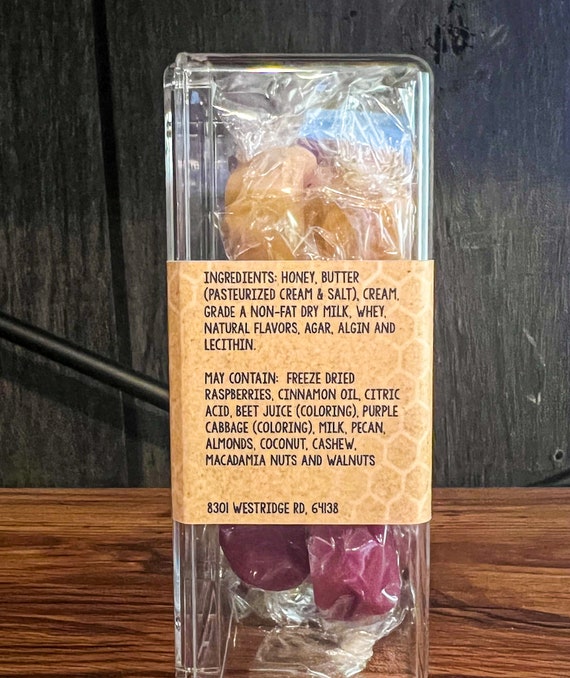The image depicts a clear, rectangular plastic container standing upright on a wooden surface with dark paneling in the background. The container is wrapped with a brown label that lists the ingredients on the back. Inside, individually wrapped items are visible, including a brown and a red object. The label details a range of ingredients: honey, pasteurized cream (butter and salt), cream, Grade A nonfat dry milk, whey, natural flavors, agar, algin, lecithin, freeze-dried raspberries, cinnamon oil, citric acid, beet juice, purple cabbage, milk, pecans, almonds, cashews, macadamia nuts, and walnuts. This suggests the contents are a healthier version of candy, emphasizing natural and nutritionally beneficial components.